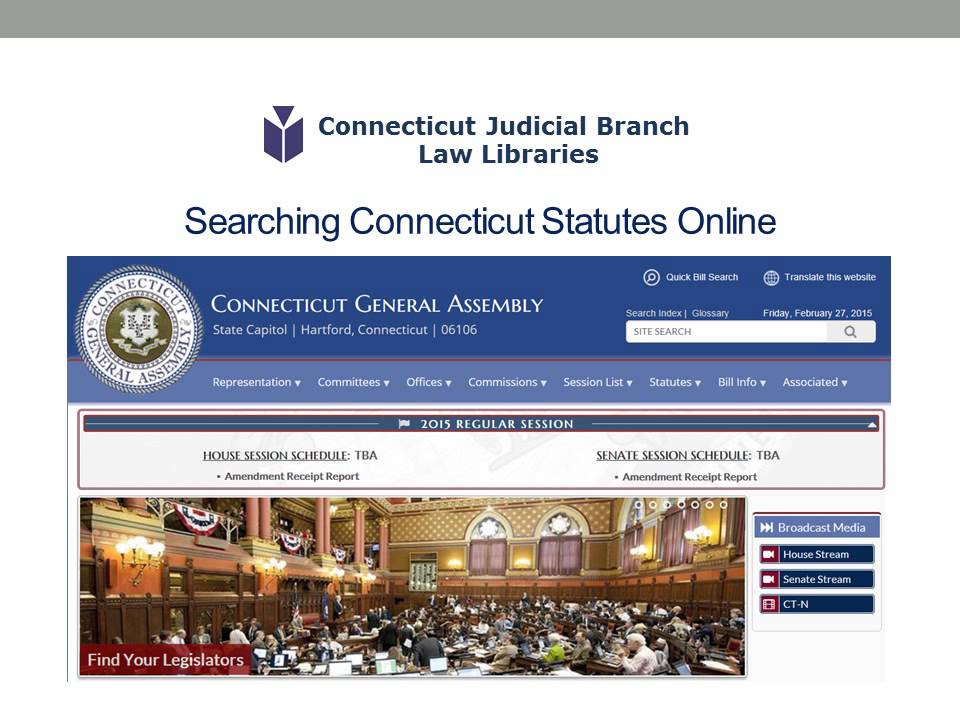A webpage displays information about the Connecticut Judicial Branch Law Libraries, prominently presented in blue text. On the left, a simple navy icon of an open book with a floating triangle above it visually represents the libraries. Below this, the heading "Searching Connecticut Statutes Online" is centered and also in blue.

Further down, an inset shows the Connecticut General Assembly website, mostly in white. It is identified with the address: "State Capitol, Hartford, Connecticut, 06106" and features the assembly's gold emblem resembling a badge. In the top right corner, options for "Translate This Website" and "Quick Bill Search" are available, followed by a general "Site Search" option. There are also details about the 2015 legislative session, indicating that the House and Senate session schedules are yet to be announced.

The embedded image shows the legislative body in session at the Capitol Hill. Key visual elements include stained glass windows and patriotic red, white, and blue banners draped over railings. The legislators are seated row by row at desks, engaged with papers. To the right, there are quick-access tabs for "Broadcast Media," "House Stream," "Senate Stream," and "CT-N."